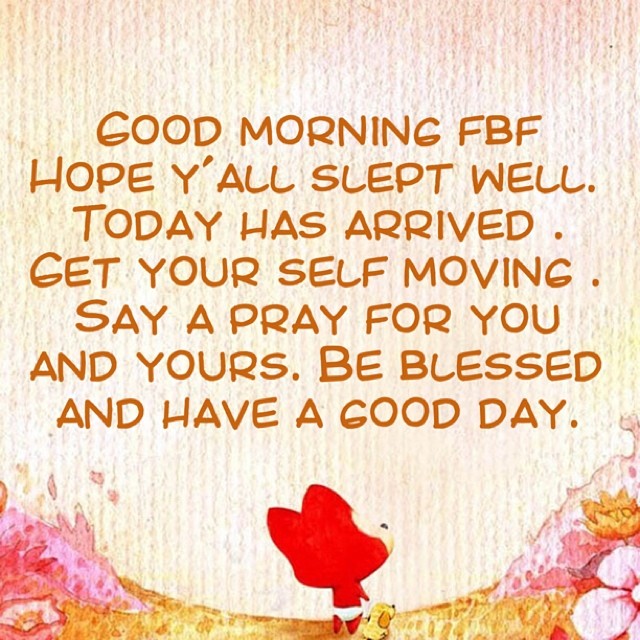The image is a print and graphic artwork that resembles a poster set against a creamy, almost pinkish golden background, akin to the texture of old paper or cardboard. It prominently features an inspiring quote in all caps, orange lettering: "Good morning FBF, hope y'all slept well. Today has arrived. Get yourself moving. Say a prayer for you and yours. Be blessed and have a good day." Below this uplifting message, there is a detailed drawing of two animals. The first is a large, fiery red fox standing upright on two legs, wearing white underwear and gazing upward at the text. Beside the fox is a much smaller yellow dog with dark brown ears and a tiny black button nose, also looking up toward the sky. The duo stands amidst a collection of pink and orange flowers, some of which are arranged in a wave-like pattern around and beneath them, creating a vibrant, almost ethereal valley-like scene.